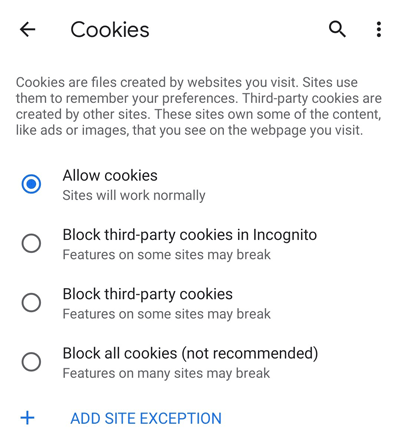The image depicts a smartphone screen displaying a web page dedicated to managing cookie settings. At the top of the screen, a header reads "Cookies" followed by a left-facing arrow. To the right of this header are a search icon and three vertical dots indicating additional options.

Beneath the header, explanatory text describes cookies as files created by websites to store user preferences. It also explains that third-party cookies are created by other sites, often containing ads or images seen on the web page being visited.

Below the descriptive text, there are a series of vertically-aligned options with radio buttons next to each:

1. The first option, "Allow cookies," is selected. The accompanying text indicates that selecting this option allows websites to function normally.
   
2. The second option, "Block third-party cookies in Incognito," is not selected. The subtext mentions that enabling this option may cause some site features to break.
   
3. The third option, "Block third-party cookies," is also not selected. Similar to the previous option, the subtext warns that site features may be impaired.

4. The fourth and final option, "Block all cookies" (not recommended), is not selected. The subtext advises that many site features could break if this option is enabled.

At the end of the page, there is a plus symbol followed by the text "Add site exception" in all capital letters, suggesting a feature for adding specific sites to an exception list regarding cookie management.

Overall, the image represents a comprehensive interface for managing cookie settings on a smartphone.